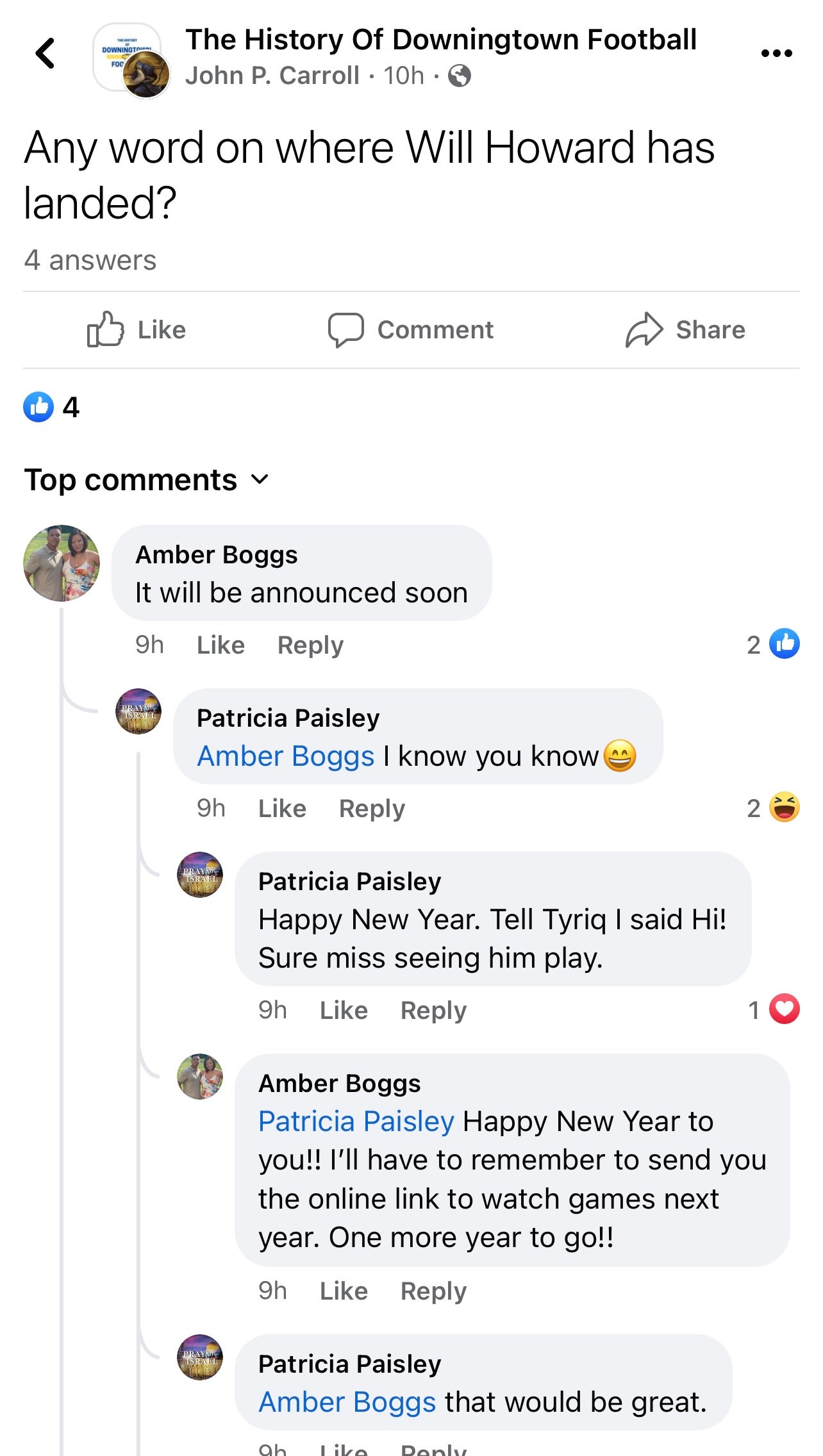The image showcases a Facebook post on the "History of Downington Football" page by John P. Carroll. The post, made 10 hours ago, features John inquiring, "Any word on where Will Howard has landed?" Below the post, there is an interaction bar allowing users to like, comment, or share.

The first comment is by Amber Boggs, who responded nine hours ago, stating, "It will be announced soon," with two likes. Patricia Paisley replied to Amber's comment with, "Amber Boggs I know you know 😊," which garnered two laugh reactions. Patricia also commented, "Happy New Year! Tell Tarek I said hi; sure miss seeing him play," accompanied by a heart emoji. Amber responded, "Happy New Year to you! I'll have to remember to send you the online link to watch games next year. One more year to go." Finally, Patricia replied, "Amber Boggs that would be great."

The layered conversation highlights an active and engaged community eagerly discussing updates and maintaining personal connections related to Downington Football.